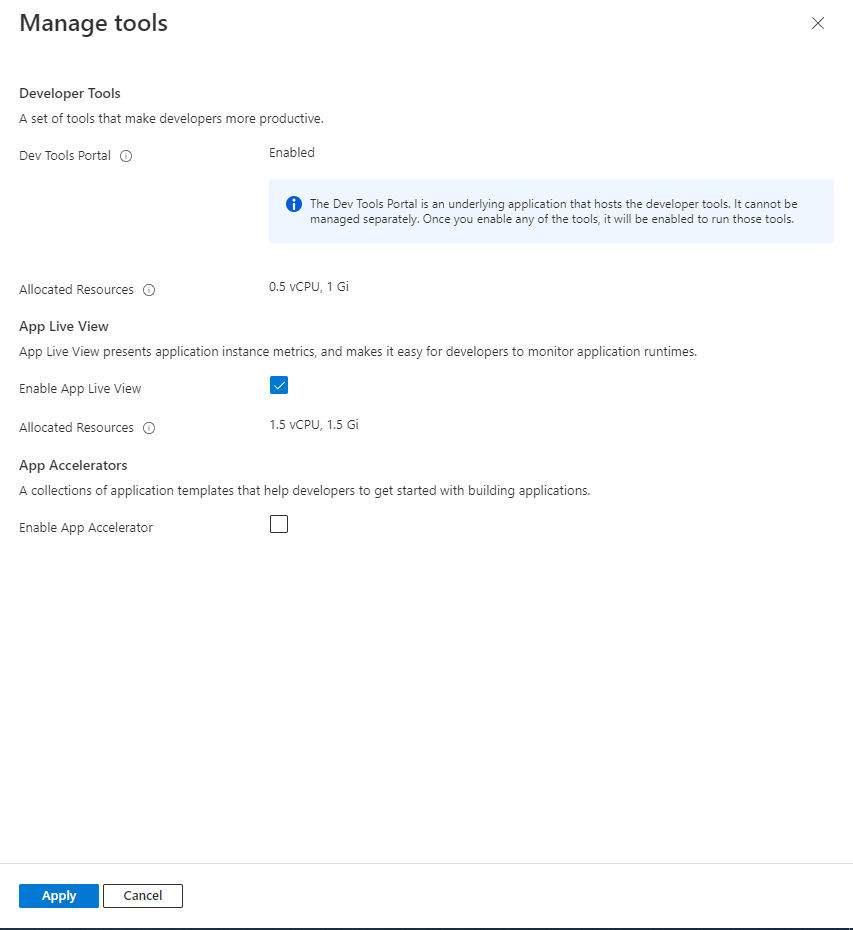In the top left corner, the text "Manage Tools" is displayed in a basic, black, somewhat bold font. Directly beneath this, in a slightly smaller size of the same font, it reads "Developer Tools" in an even smaller size. Below this heading, the text explains, "A set of tools that make developers more productive." 

Next comes the heading "DevTools Portal," accompanied by a small circular icon containing an eye, indicating that additional information is available upon hovering. To the right, the text "Nexus enabled" appears, followed by a rectangular notification bubble with a light blue background. This bubble includes a dark blue eye icon with a white center and a small black font description that reads, "The DEVTools Portal is an underlying application that hosts the developer tools. It cannot be managed separately. Once you enable any of the tools, it will be enabled to run those tools."

Further down, the text "Allocated Resources" accompanied by the eye symbol, specifies the resources allocated as "0.5v CPU, 1Gi." 

In bold lettering, "AppLiveView" is presented. Underneath this heading, in non-bold text, it explains, "AppLiveView presents application instance metrics and makes it easy for developers to monitor application runtimes." Below this description, the option "Enable AppLiveView" is displayed, alongside a checkbox that is ticked, indicated by a dark blue background with a white checkmark inside. 

Further down, the text "Allocated Resources" appears again with the eye symbol, indicating "1.5v CPU, 1.5Gi."

In bold text, the heading "AppAccelerators" is presented. Beneath this, in non-bold text, it explains, "A collection of application templates that help developers to get started with building applications."